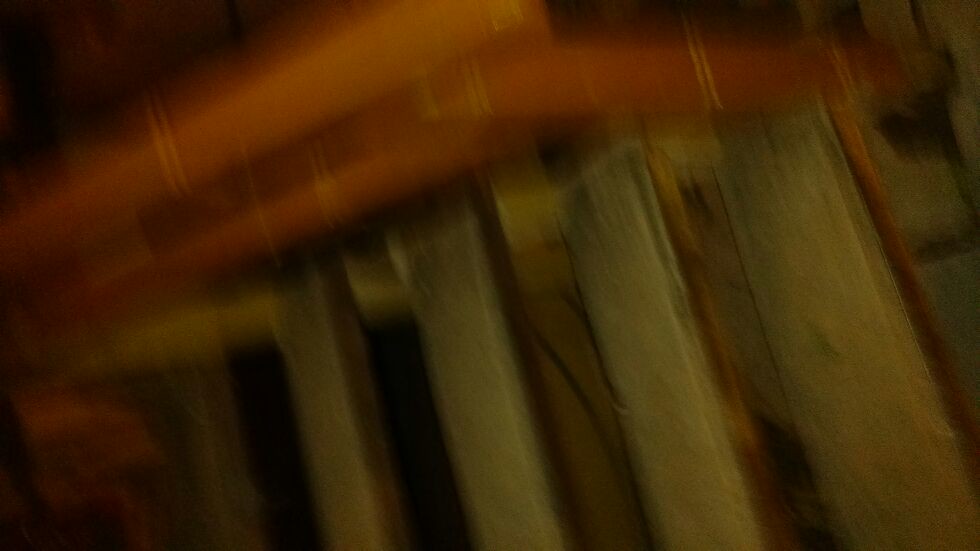This extremely blurry and likely accidental photo appears to depict a wooden staircase with a dark stained handrail, viewed from an extreme angle, possibly sideways. The stairs feature open slats and there are five steps visible. To the side, there's a section of red brickwork partially illuminated by light from the top of the image, while the bottom remains dark. The upper right corner shows a small wooden area, reinforcing the impression of it being a staircase rather than pillars or an overhang. Elements of light and various colors contribute to the chaotic mishmash, making it difficult to determine the exact scene.